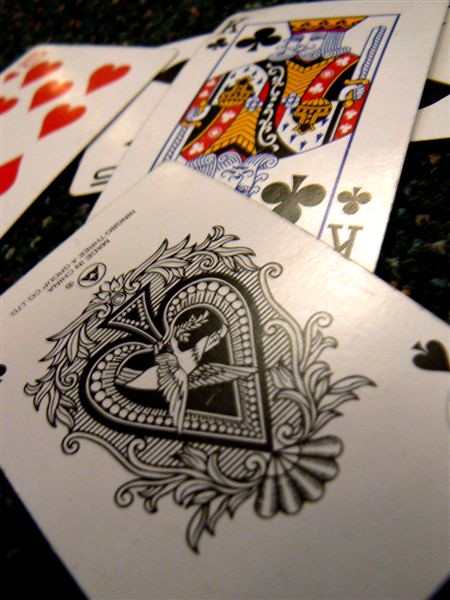This image showcases a detailed arrangement of playing cards set against a textured black background adorned with colorful threads. Dominating the foreground is an Ace of Spades, notable for its intricate design featuring an eagle majestically perched in the center of the large spade symbol. The spade itself is outlined with what appear to be pens, pencils, or logs meticulously stacked on top of one another, and is further embellished with decorative garlands.

Above the Ace of Spades, there is a King of Clubs, rendered in the classic style of standard face cards. The king is depicted holding a sword in each hand, with the swords oriented in opposite directions, creating a mirrored but reversed effect.

Partially visible beneath the King of Clubs is the Ten of Spades, identifiable by the black spade symbols despite its limited visibility. Superimposed on the corner of the Ten of Spades is the clearly visible Ten of Hearts.

The black background provides a striking contrast to the playing cards, with its colorful threads or sections woven into the material, adding depth and texture to the scene.